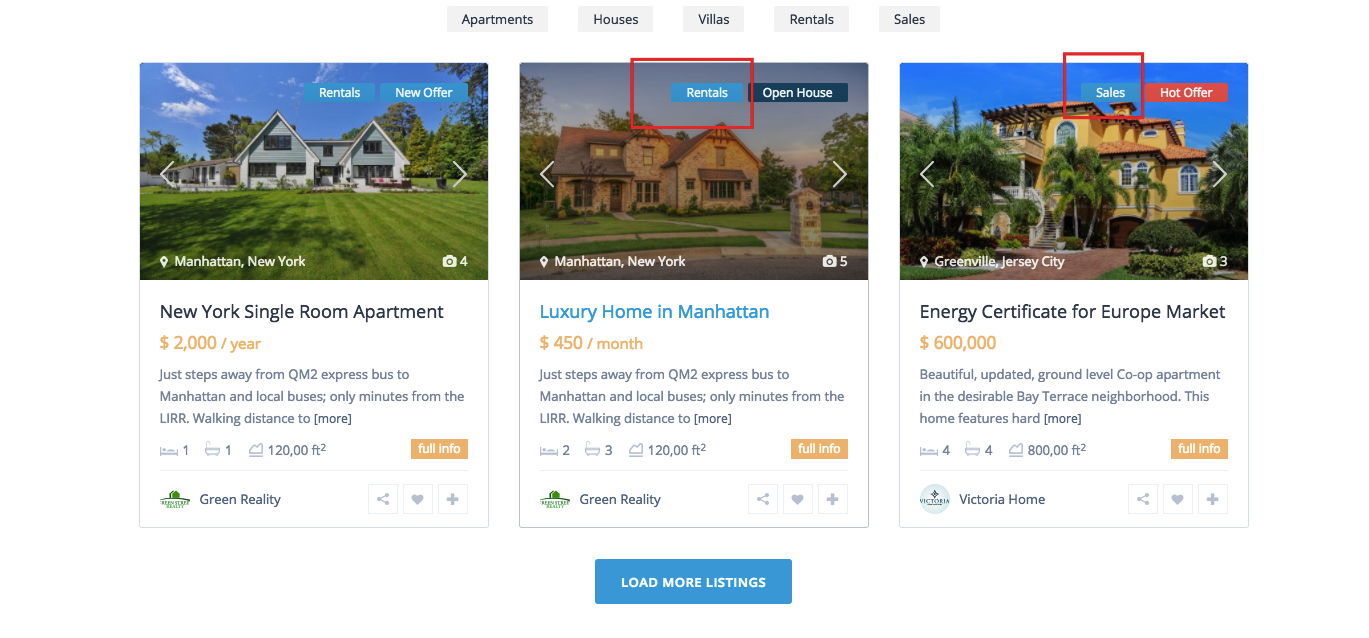A left-to-right horizontal image showcases a phone search interface set against a plain white background, likely provided by the user's computer screen. The interface, which can be accessed through a smart device or webpage, features a set of gray rectangular tabs at the top center of the screen. Each tab is labeled in black text with clickable options: "Apartments," "Houses," "Villas," "Rentals," and "Sales."

Beneath these tabs, there are three vertical sections displaying properties with accompanying images and detailed information:

1. **First Property**: Located in Manhattan, New York, this listing falls under the "Rentals" category and is marked as a "new offer." The property is a single-room apartment priced at $2,000 per year. It includes four photos and highlights its proximity to public transportation, being just steps away from the QM2 Express bus to Manhattan, local buses, and walking distance to the LIRR. The listing promises more detailed information via a clickable option and is managed by *Green Realty*.

2. **Second Property**: Also in Manhattan, New York, this rental is available for $450 a month and is designated as an "open house." Described as a luxury home, the listing is similarly close to the QM2 Express bus to Manhattan, local buses, and the LIRR. The property is clearly demarcated with a red box around the word "Rentals," and additional information can be accessed by clicking on another option. This listing is also managed by *Green Realty*.

3. **Third Property**: This listing is labeled under "Sales" as a hot offer priced at $600,000. It pertains to an "energy certificate for your market," provided by *Victoria Home*. The listing includes a brief description and detailed information is available upon request.

Overall, the image effectively presents a clean and organized layout for browsing real estate options with clear, accessible details for potential renters or buyers.